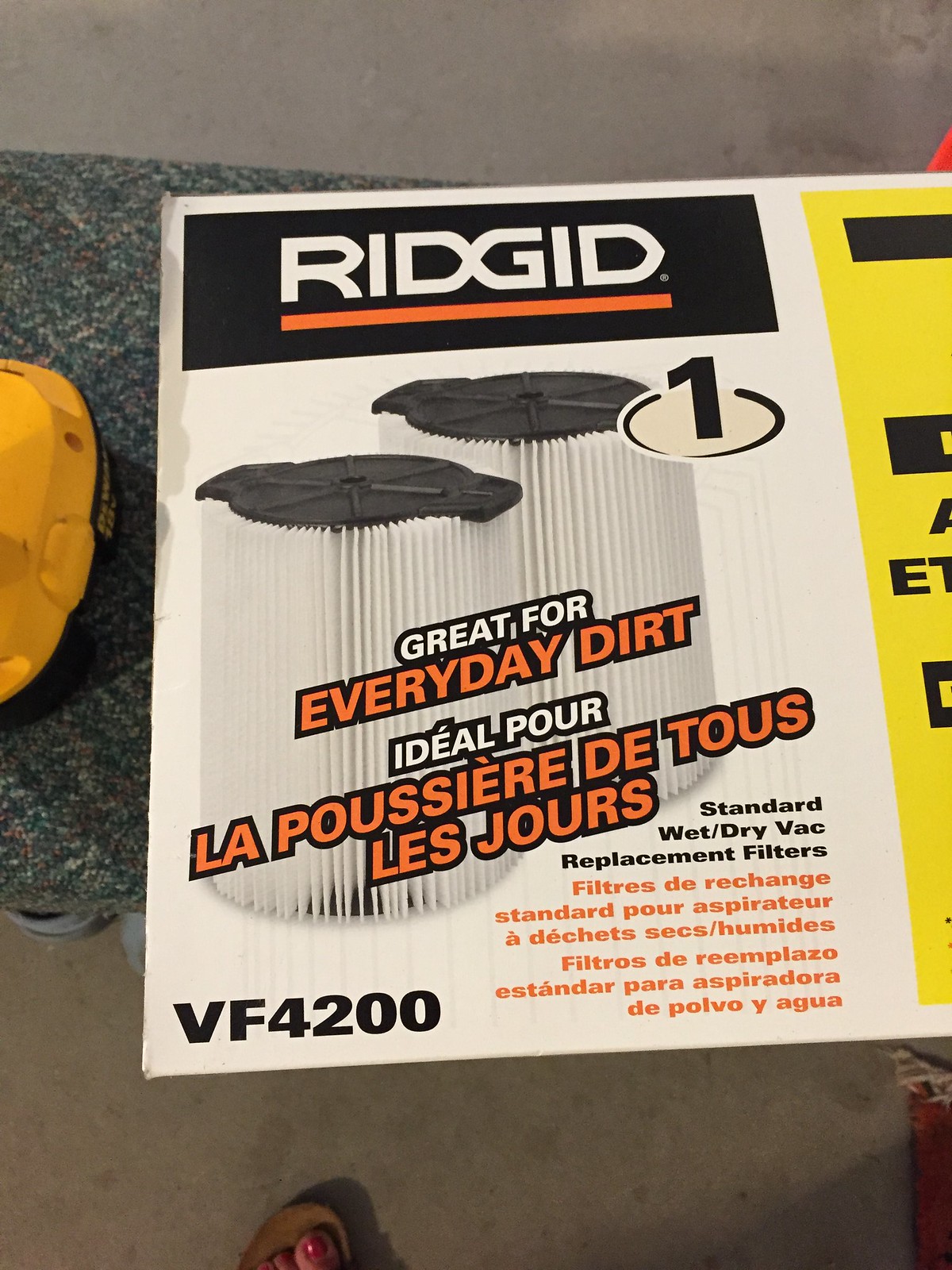The image captures a detailed advertisement for R-I-D-G-I-D standard wet/dry vacuum replacement filters, likely from a magazine or product instructions. It is positioned on a work surface, with part of an orange device visible to the left and a cement floor beneath, showing a woman's red-painted toes in open-toe sandals.

The advertisement occupies a predominantly white background, divided by a thick black border at the top with "R-I-D-G-I-D" written in bold white letters underlined in orange. Below this header are two vertically oriented, round filters featuring a white channeling design and black tops. To the upper left is the text "Great for everyday dirt," displayed in both English and French, with "Great for" in white and "everyday dirt" in orange. Additional text indicates these are "Standard wet/dry vac replacement filters," with the English version in black and another translation, likely French or Spanish, in orange below. The model number VF4200 is situated in the lower left corner in a black font. The right side of the advertisement features a partial view of a yellow background adorned with bold, black text that is partially cut off.